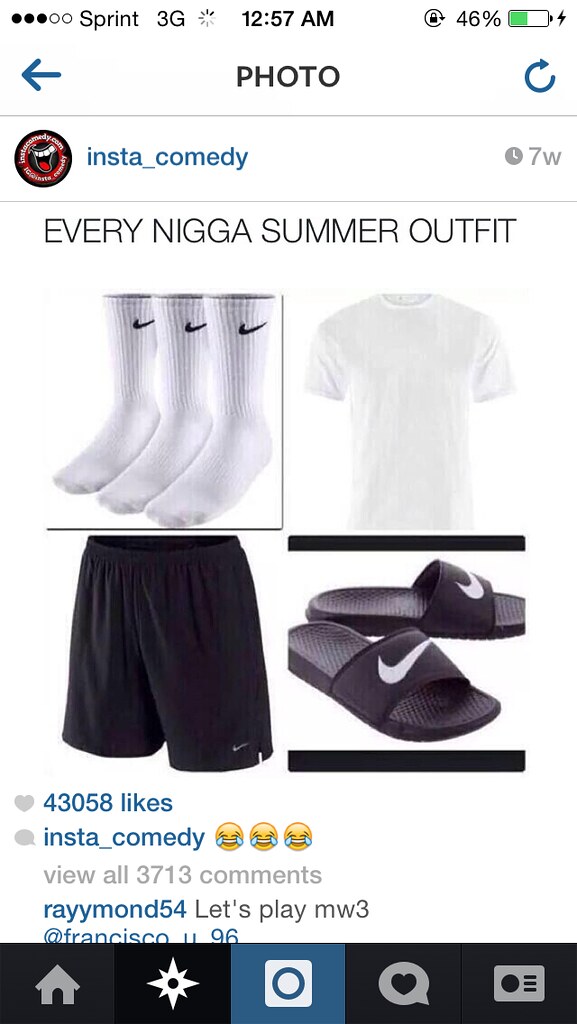This is a detailed screenshot of an Instagram page captured from a mobile phone. The background of the image is predominantly white. At the very top of the screenshot, there are five dots indicating signal strength, with three black dots and two white ones, followed by the network details "Sprint 3G." Further to the right, it displays the time as 12:57 AM, a lock icon, and a battery indicator showing 46% power with a green half-filled battery icon. There's an arrow pointing left on the leftmost corner, and a refresh button on the rightmost corner under the header "Photo."

Below this, there's a horizontal strip bordered by gray lines. On the left is a logo for InstaComedy, depicting an open mouth with white teeth and a red tongue, along with the text "instacomedy.com." Next to it is the page name "insta_comedy." On the right side of this strip, there is a clock icon next to the text "7W," indicating the post age.

Underneath, a bold text reads "Every Nigga Summer Outfit," showing a collage of four images: three white Nike socks, a white round-neck t-shirt, black shorts, and black Nike flip-flops. Below the collage, it states "43050 likes" alongside a gray heart icon.

Further down, a speech bubble feature includes the page name "instacomedy" followed by three laughing emojis. This is accompanied by the text "View all 3713 comments." Below this, a comment from "Raymond54" reads "let's play MW3," tagging "FranciscoU96."

At the bottom, there is a black strip containing navigation buttons: a home icon, a star icon, an Instagram icon, a comment icon with a heart, and a camera icon.